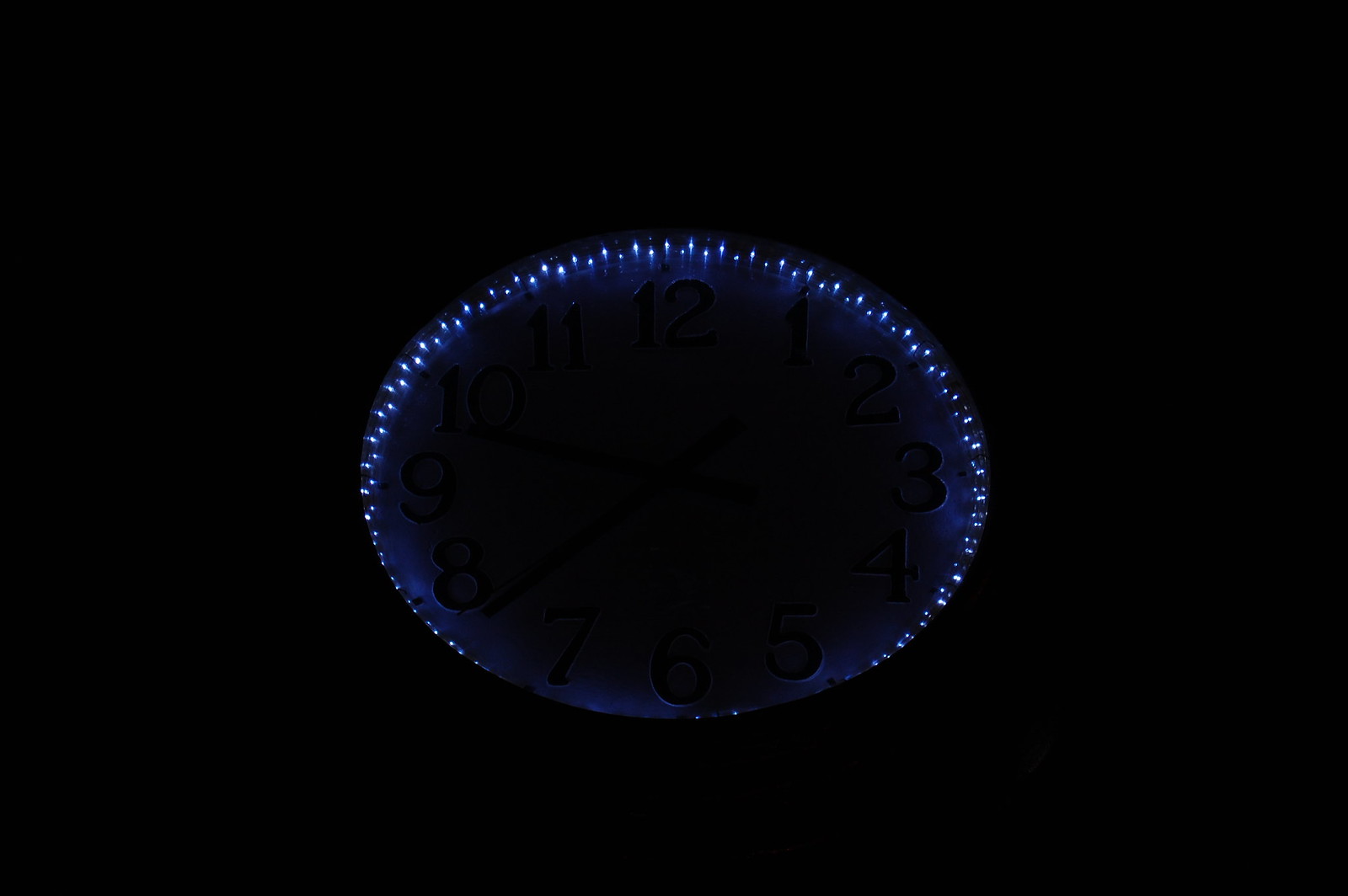The image features a clock with a pitch-black background, making it difficult to discern precise details. The clock face is faintly illuminated by a ring of small, bluish-white LEDs neatly arranged around its outer edge. These lights create a soft blue glow that highlights the clock’s perimeter and faintly outlines the raised numbers from 1 to 12 in their usual positions. The LEDs are evenly spaced and cast minimal shadows inward towards the center of the clock. The time displayed is approximately 9:38. Although the glow provides minimal illumination to the clock’s surface, it is insufficient to reveal any other elements or details prominently, leaving much of the image obscured in darkness.